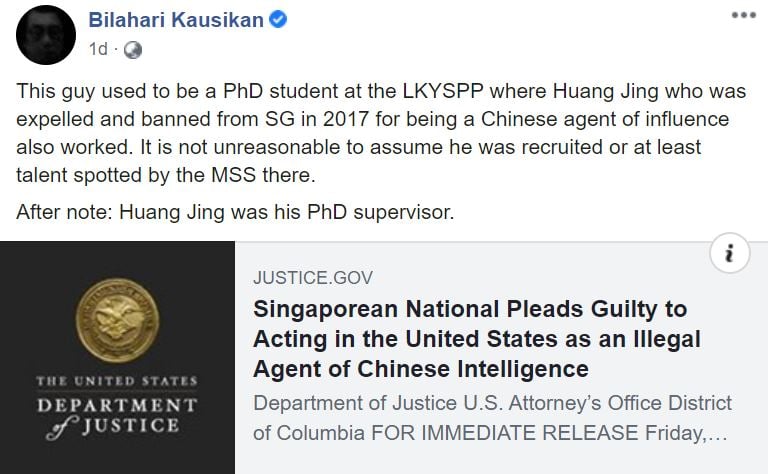The image shows a Facebook post by Bilahari Kausikan, who is verified by a blue checkmark next to his name. To the left of the username is a black-and-white photograph of Bilahari's face, although the image is quite dark. The post was made one day ago. In the post, Bilahari comments: "This guy used to be a Ph.D. student at the LKYSPP, where Huang Jing, who was expelled and banned from SG in 2017 for being a Chinese agent of influence, also worked. It is not unreasonable to assume that he was recruited or at least talent spotted by the MSS there. After note, Huang Jing was his Ph.D. supervisor." 

Below this text, there is a link to a Justice.gov website. The linked article's headline reads: "Singaporean National Pleads Guilty to Acting in the United States as an Illegal Agent of Chinese Intelligence." Accompanying this headline is the beginning text of the article, an information bubble to the upper right, and an image of the United States Department of Justice seal to the left.